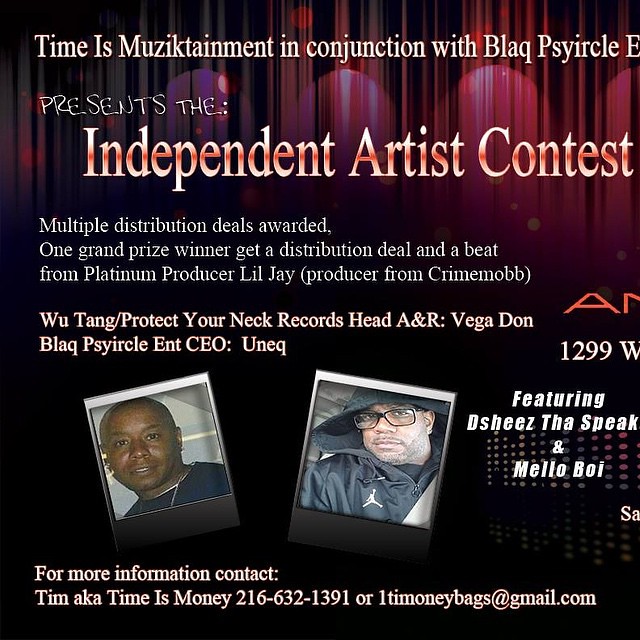The image is a text-based graphic design advertising the "Independent Artist Contest." The top part features a slightly whitish-yellow font that reads, "Time is Musictainment in conjunction with Black Cyrical," though part of this text is cropped out. Below that, in a spray-paint font, it says, "Presents The." The main title "Independent Artist Contest" is boldly displayed in a large font that's a mixture of white and red. Underneath, in white font, it announces, "Multiple Distribution Deals Awarded. One Grand Prize Winner gets a distribution deal and a beat from Platinum Producer Lil' J (Producer from Crime Mob)." Further down, the text includes, "Wu-Tang/Protect Your Neck Records Head A&R, Vegadon; Black Cyrical Ent. CEO, Uneq (U-N-E-Q)." 

At the bottom center of the image, there are photographs of two African-American men. The man on the left wears a dark blue t-shirt and is bald, looking directly at the camera. The man on the right has black-framed glasses, a black hat or hoodie featuring the Jumpman Nike Michael Jordan logo. To the right of these images, although somewhat cropped, the text mentions, "1299W Featuring Dee Shees, The Speak, and Mellow Boy." 

The background transitions from a stage curtain mixture of red and black at the top, to a solid black at the bottom where the text, "For More Information Contact Tim, AKA Time Is Money, 216-632-1391, or 1TimMoneyBags@gmail.com," is displayed.